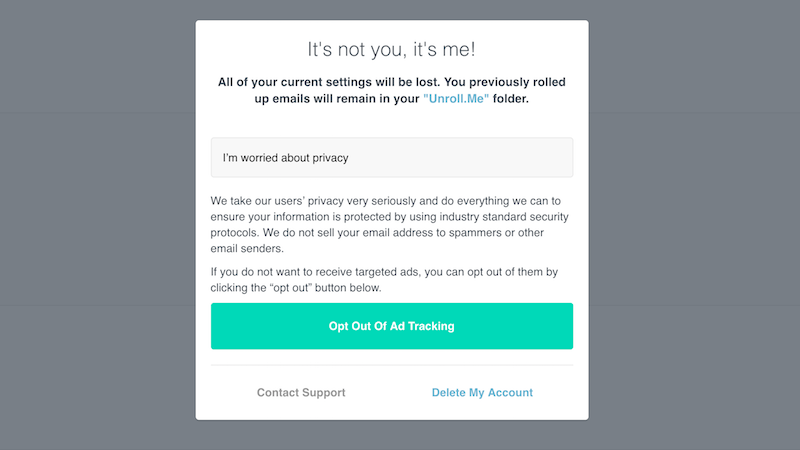The image depicts a webpage related to account management, likely from a service that helps manage email subscriptions. The main message at the top of the image reads, "It's not you, it's me. All of your current settings will be lost." This suggests the user is in the process of altering or deleting their account settings. It also mentions that previously rolled-up emails will remain in the "Unroll Me" folder, indicating this service's specific feature.

A section addressing privacy concerns states, "We take our user's privacy very seriously, and do everything we can to ensure your information is protected by using industry-standard security protocols. We do not sell your email address to spammers or other email senders." Below this message, there is an option to opt out of targeted ads, with a corresponding button labeled "Opt-out of ad tracking," which has a green background and white text.

At the bottom of the page, two additional options are presented: a "Contact Support" button in gray and a "Delete My Account" button in blue. The text throughout the page is primarily black on a white background, with buttons mainly in green and blue. The page has a darker gray border, which contrasts subtly with the white content area, making the border stand out slightly. Overall, the layout and style of the page are typical of web interfaces designed for managing account settings or initiating account deletion.